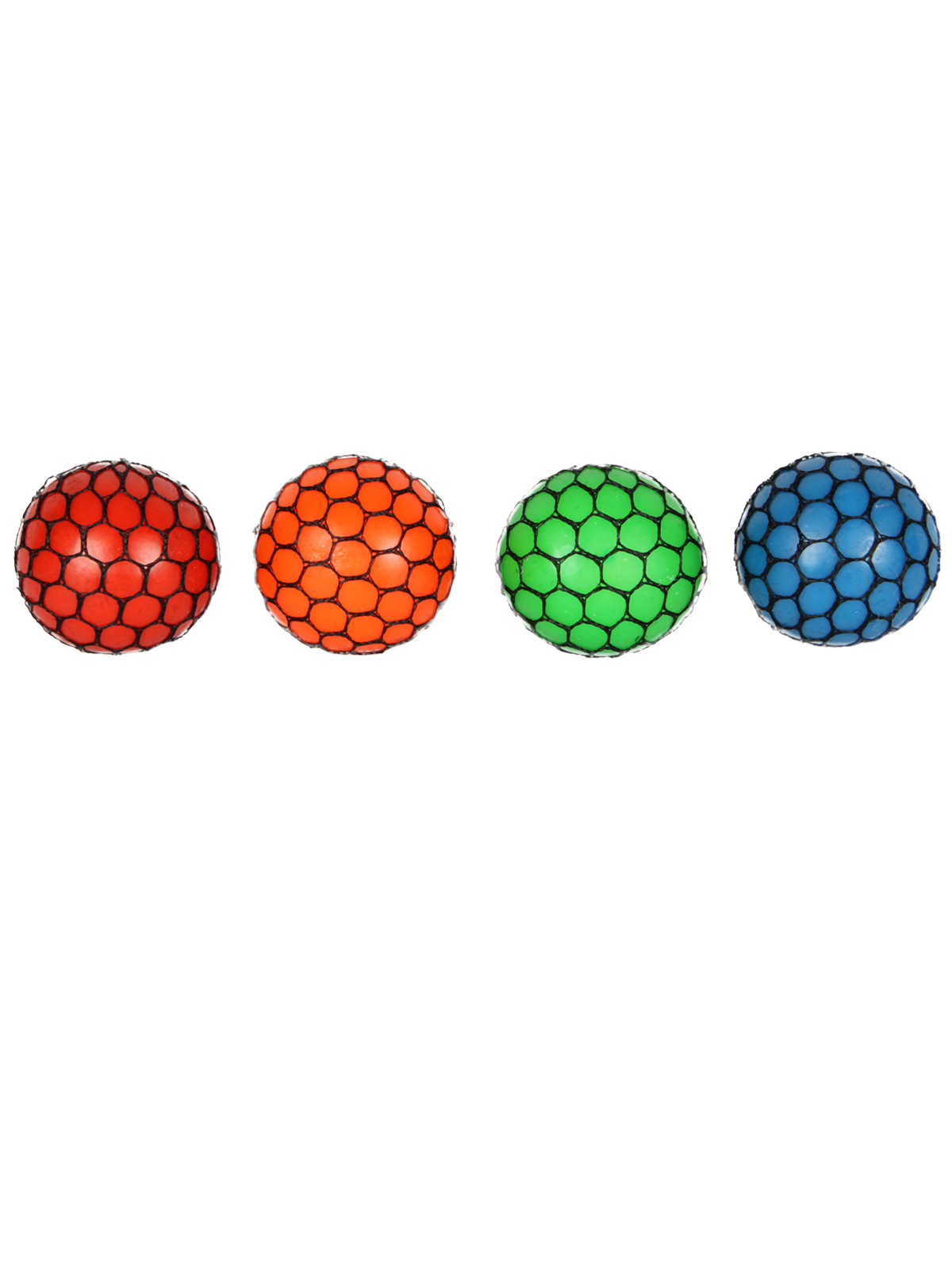This image showcases four small gym or exercise balls, each adorned with a distinctive black honeycomb netting. The balls are arranged in a horizontal line with no background, creating a floating effect against a white transparent backdrop. From left to right, the colors of the balls are red, orange, green, and a darker blue. The absence of any text or description in the image allows the vibrant colors and unique geometric pattern of the black netting to stand out clearly.